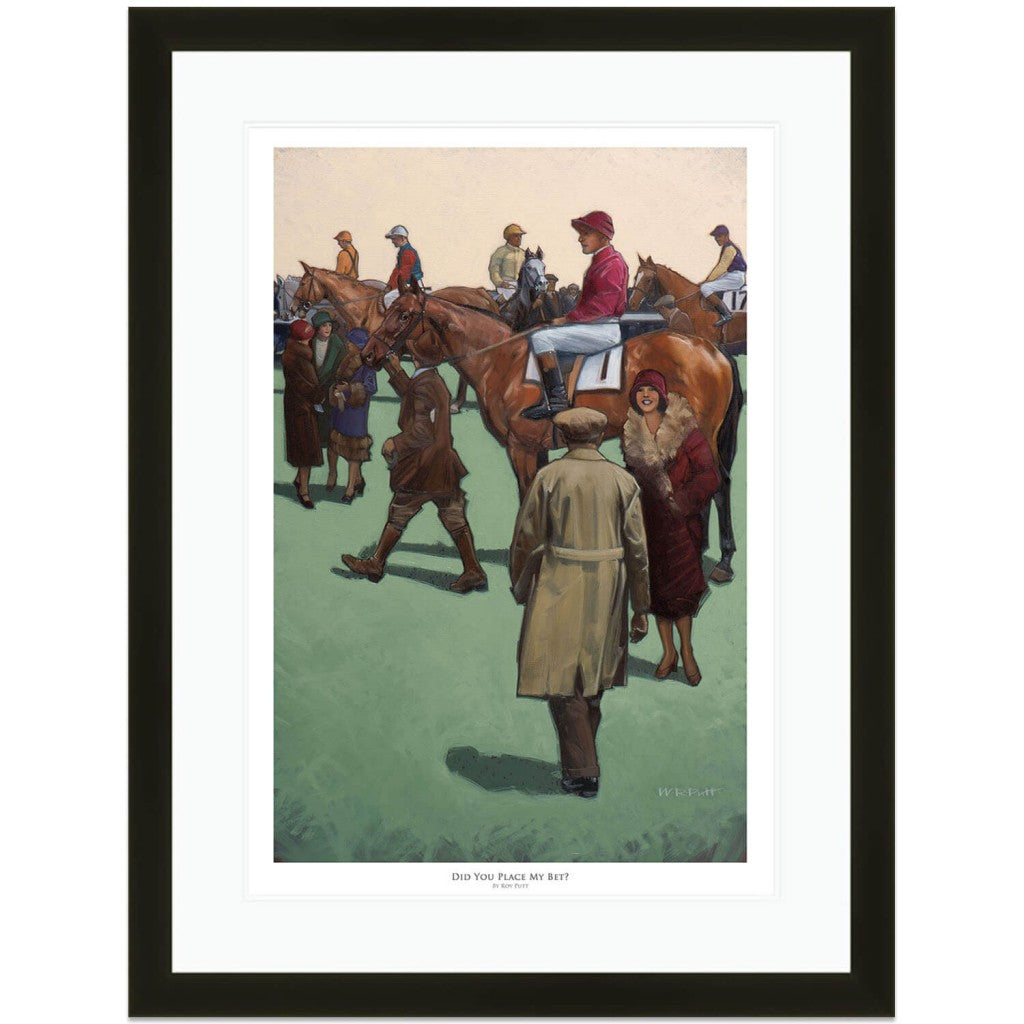This framed painting, which is in portrait orientation and bordered by a heavy black frame with a white mat, vividly captures a pre- or post-horse race scene. The caption at the bottom center reads, "Did you place my bet?" in black text, with smaller, unreadable text beneath it. The central focus is a jockey on a brown horse, both facing left. The jockey is dressed in a maroon shirt and cap, white pants, and black boots, with the number one displayed on the saddle blanket. 

In the lower right foreground, a woman in a maroon jacket with a fur collar and matching hat smiles and looks up, likely at the man approaching her. This man, walking toward the horse, wears a beige trench coat, a matching beret, and dark trousers. To the left of the horse, another man in a brown jacket, hat, boots, and tan pants firmly grips the horse's bridle, guiding it forward. The background showcases several other jockeys on their horses, enhancing the bustling, anticipatory atmosphere of the scene. The ground cover in the foreground is a light aqua, contrasting with the cream-colored sky above. The overall style of the artwork is distinctly equestrian, celebrating the spirited world of horse racing.